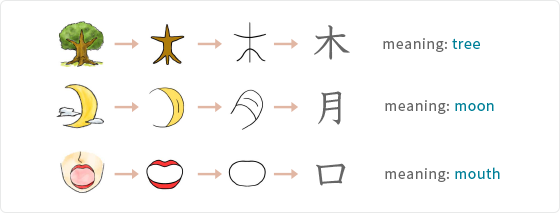The image is a horizontally rectangular diagram with a thin light gray or light blue border on a white background, resembling a Rosetta Stone for learning Japanese characters. It is divided into three rows, each showing a sequence that transitions from a colorful picture to the corresponding Japanese kanji.

The top row features a brown tree with green leaves, followed by an arrow pointing to just the brown trunk, then another arrow leading to a simple line drawing of the trunk. This sequence progresses to a bold green kanji character, with the annotation "meaning: tree" in black and blue text.

In the middle row, there is an illustration of a yellow crescent moon with white clouds. The following image isolates the crescent moon, which then transitions through an arrow to a line drawing resembling its shape. The final image in this row is a darker black kanji character, annotated with "meaning: moon."

The bottom row displays a cartoon face from the nose down with an open pink mouth and red lips. The sequence continues with an arrow pointing to just the red lips, another arrow to an oval shape, and finally to a square kanji character, labeled "meaning: mouth."